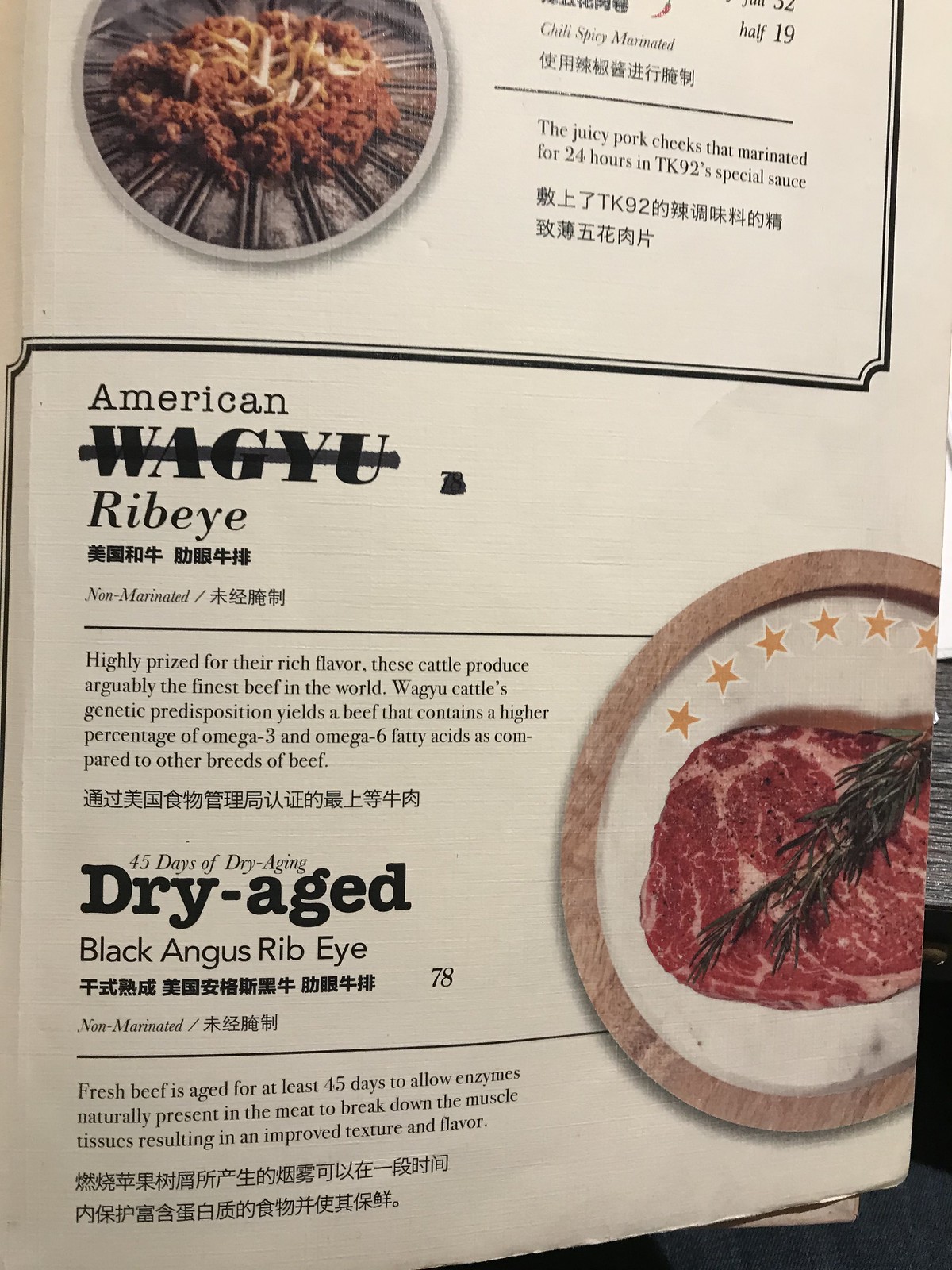This is a photograph of a portion of a menu, predominantly in an Oriental language with English translations. The upper part of the page showcases a circular plate featuring a dish described as "chili, spicy, marinated, the juicy pork cheeks that have been marinated for 24 hours in TK-92's special sauce." The plate appears to have a distinct design with projections resembling spokes. Encircling this description, there are Chinese characters. Below, the menu lists "American Wagyu ribeye, non-marinated," highlighting its rich flavor and superior qualities due to the Wagyu cattle's genetic predisposition for higher omega-3 and omega-6 fatty acids. To the right, there is an image of an uncooked steak with a sprig of basil on top. Lastly, the menu details a "45 days dry-aged Black Angus ribeye," priced at $78.00. This section also features Chinese text and an image of the ribeye steak on a plate.